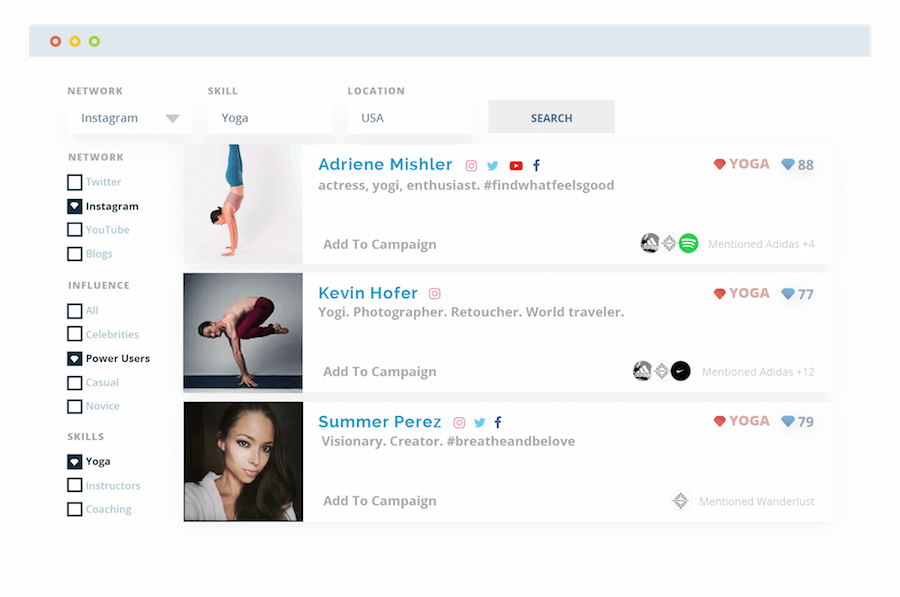This is a detailed screenshot from an Apple product, displayed in landscape orientation, featuring a white background. At the top, there's a characteristic gray bar with the familiar red, yellow, and green hollowed-out circles indicative of a Mac OS window. Beneath this bar lies a clean, white space populated with various interface elements.

The main interface is divided into columns labeled "Network," "Skill," and "Location," each with corresponding drop-down menus. The "Network" menu is set to "Instagram," the "Skill" menu to "Yoga," and the "Location" menu to "USA." Adjacent to these menus, a prominent search button invites user interaction.

Under the "Network" column, you’ll find multiple social media platforms available for selection, including Twitter, Instagram, YouTube, and Blogs. The "Influence" section allows users to filter based on categories like All, Celebrities, Power Users, Casuals, and Novices. For skills, you can select options like Yoga, Instructors, and Coaching.

The results section provides detailed profiles of influencers. The first profile features Adrienne Mishler, depicted doing a handstand, accompanied by some personal information. Following her is Kevin Hoffer, shown balancing on his hands with his legs elevated, along with more details about him. Lastly, Summer Perez's profile is displayed with an image of her gazing intently, hair parted to the side, along with additional information.

Overall, this screenshot illustrates a sophisticated and user-friendly interface designed to filter and display influencer data based on specified criteria.